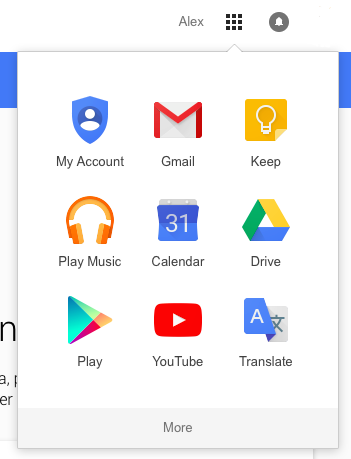The image is set against a white background featuring a centered grey font displaying the name "Alex." Adjacent to the name on the right are nine small square dots arranged in a three-by-three grid. To the far right, there's a grey circle that encapsulates a white bell icon.

Below this section is a series of icons and descriptions spread across multiple rows, with each row containing several images and captions. Starting with the top row:

1. A blue shield icon featuring a white face and shoulders, accompanied by the text "My Account."
2. To its right, a red "M" with a grey background and the word "Gmail" underneath.
3. Further to the right, an orange square with a white light bulb outline, labeled "Keep."

The next row includes:

1. An icon resembling orange and yellow headphones, labeled "Play Music."
2. A blue box with a white "31" and some grey shading above it, titled "Calendar."
3. An icon with a blue, orange, and green triangular shape, labeled "Drive."

The subsequent row features:

1. An upside-down triangle icon in teal, red, orange, and light green colors, labeled "Play."
2. A reddish rounded square with a white right-pointing triangle inside, titled "YouTube."
3. A folded square icon with a blue "A" on top and a grey box on the bottom, labeled "Translate."

Finally, at the bottom, a grey box centered beneath in the middle of the image contains the text "More" in grey font.